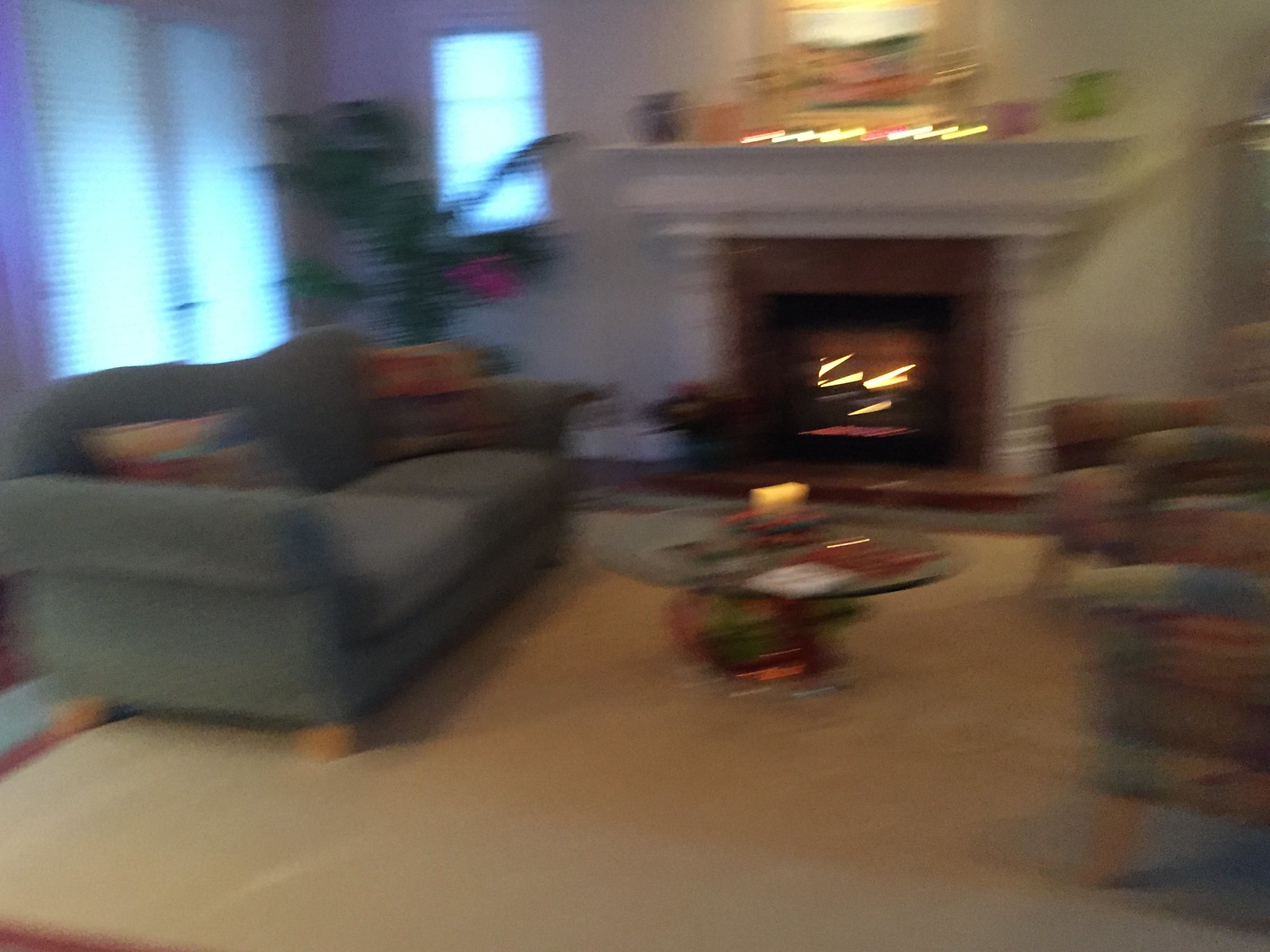This photograph showcases a charming and luxurious living room, indicative of an upscale, older home. The room exudes elegance with its massive, ornate fireplace mantle, intricate patio door design, and classic double doors, characteristic of a timeless architectural style. The room features a large, plush carpet and high-quality overstuffed furnishings, including a detailed Davenport with numerous stuffed pillows and a matching armchair to the right.

In the room, an individual is seated in a chair, though their presence is only partially visible, as the entire image is out of focus. The blurriness suggests the camera was in motion when the photo was taken, resulting in distorted and extended outlines of the objects.

Above the magnificent mantle, miniature lights subtly illuminate the space, along with a mirror or potentially a work of art that is highlighted by a spotlight. The mantle is tastefully adorned with potted flowers, adding a touch of natural beauty. In the background, double doors frame the couch, enhancing the room's grandeur. A large, potted fern occupies one corner, contributing to the lush atmosphere.

A round coffee table is centrally placed, but the objects on its surface are indiscernible due to the photograph's blurry nature. Despite the distortion, the luxurious and meticulously decorated essence of this beautiful living room is unmistakable.